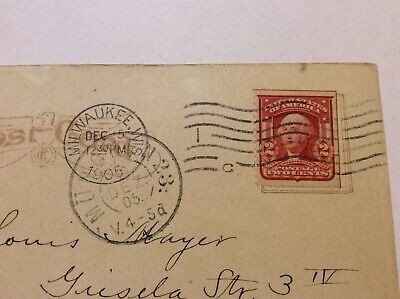This is an old, somewhat grainy photograph of the top right corner of a weathered yellow envelope, which has possibly been repurposed into a postcard. The photograph, framed in a light pink to purple backdrop, measures approximately three inches wide by just under three inches high. Dominating the top right corner of the envelope is a red postage stamp featuring an image of an individual resembling George Washington, flanked by the number two and inscribed with "United States of America" at the top and "Ten Cents" at the bottom. The stamp is marked with black wavy cancellation lines, indicating it has been postally used. Beside the red stamp are two circular ink stamps; one clearly reads "Milwaukee, December 5th, 1905," while the other, partially legible, reads "B4-5A." In the vicinity of these stamps, additional handwritten elements can be seen in black cursive pen, including a partial address: "Louise Mayer, ...GRISELA Street, 3," concluded with a Roman numeral III.